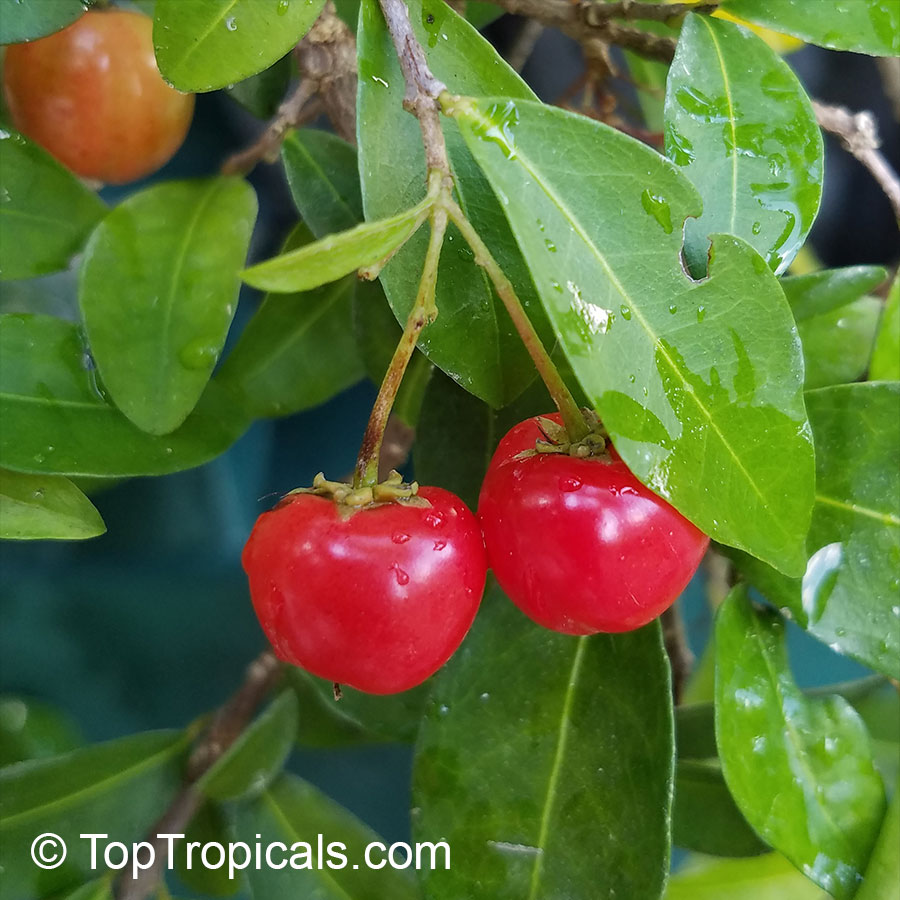The close-up photograph captures a lush section of a tomato plant outside, covered with glistening droplets of water possibly from a recent rain. Dominating the center are two small, vibrant red tomatoes, beautifully illuminated as they hang from slender green stems that branch out from a sturdy brown stem. This main stem is surrounded by an array of green leaves, some of which extend into the background, adding depth and texture to the image. In the top left corner, a tomato transitioning from green to a lighter shade of red signals its coming ripeness. Various shades of green, red, and touches of brown create a vibrant palette. The bottom left corner of the image contains white text reading "copyright toptropicals.com," hinting at the photograph's origin. Notably, one large leaf in the foreground shows signs of being nibbled on, adding a touch of nature's imperfection to the scene. The overall impression is a richly detailed glimpse into the thriving life of a tomato plant.